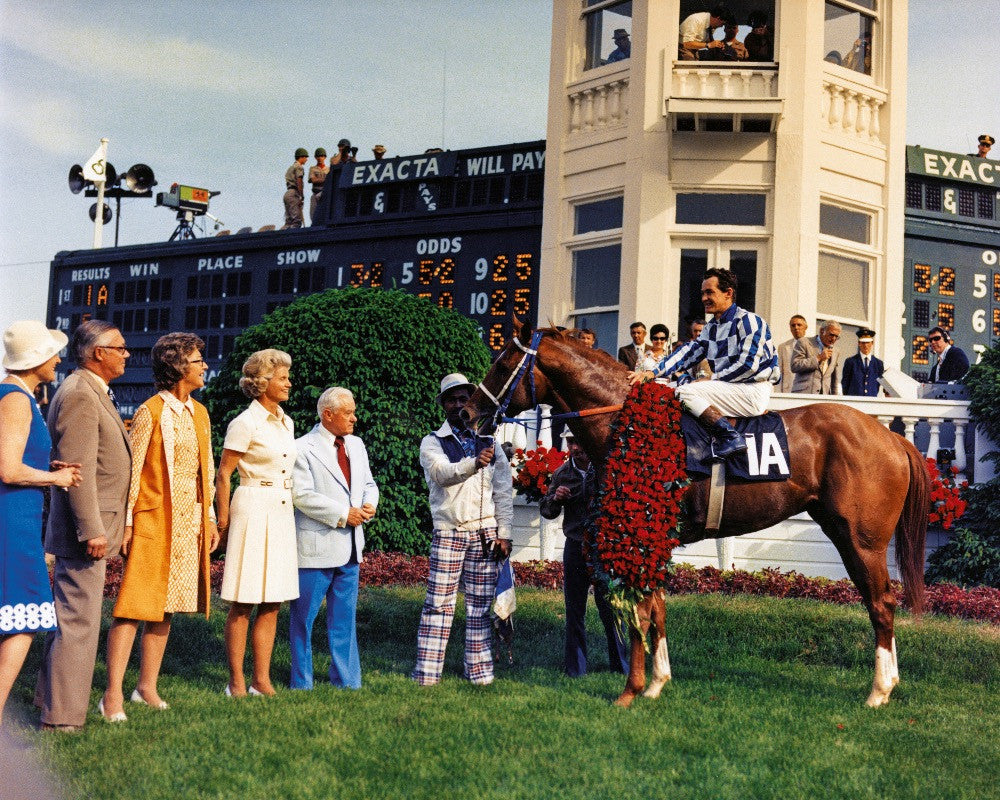A nostalgic black-and-white photograph captures a triumphant moment at a racetrack, likely from the 1960s or 70s. In the center, a well-groomed, muscular brown horse stands proudly draped in a large, ornate flower garland, signifying its victory. The jockey, identifiable by white pants and a blue-and-white striped shirt, remains seated atop the horse. Close by, a handler holds the horse's reins. To the left, six older individuals, possibly in their 50s or 60s and dressed in old-fashioned attire, stand on a patch of green grass, facing the horse in awe. Behind them, the racetrack's black wall prominently features a scoreboard listing categories like "Win," "Place," "Show," "Odds," and "Exacta." The scene is bustling, with additional spectators visible both behind a railing on the right side and around the tall, tan building in the background. This building, though partially cut off at the top, includes a tower and balcony area, likely occupied by photographers and announcers. Loudspeakers and a camera indicate the significance of the event, as the jubilant image immortalizes a horse's moment of victory in the winner's circle.